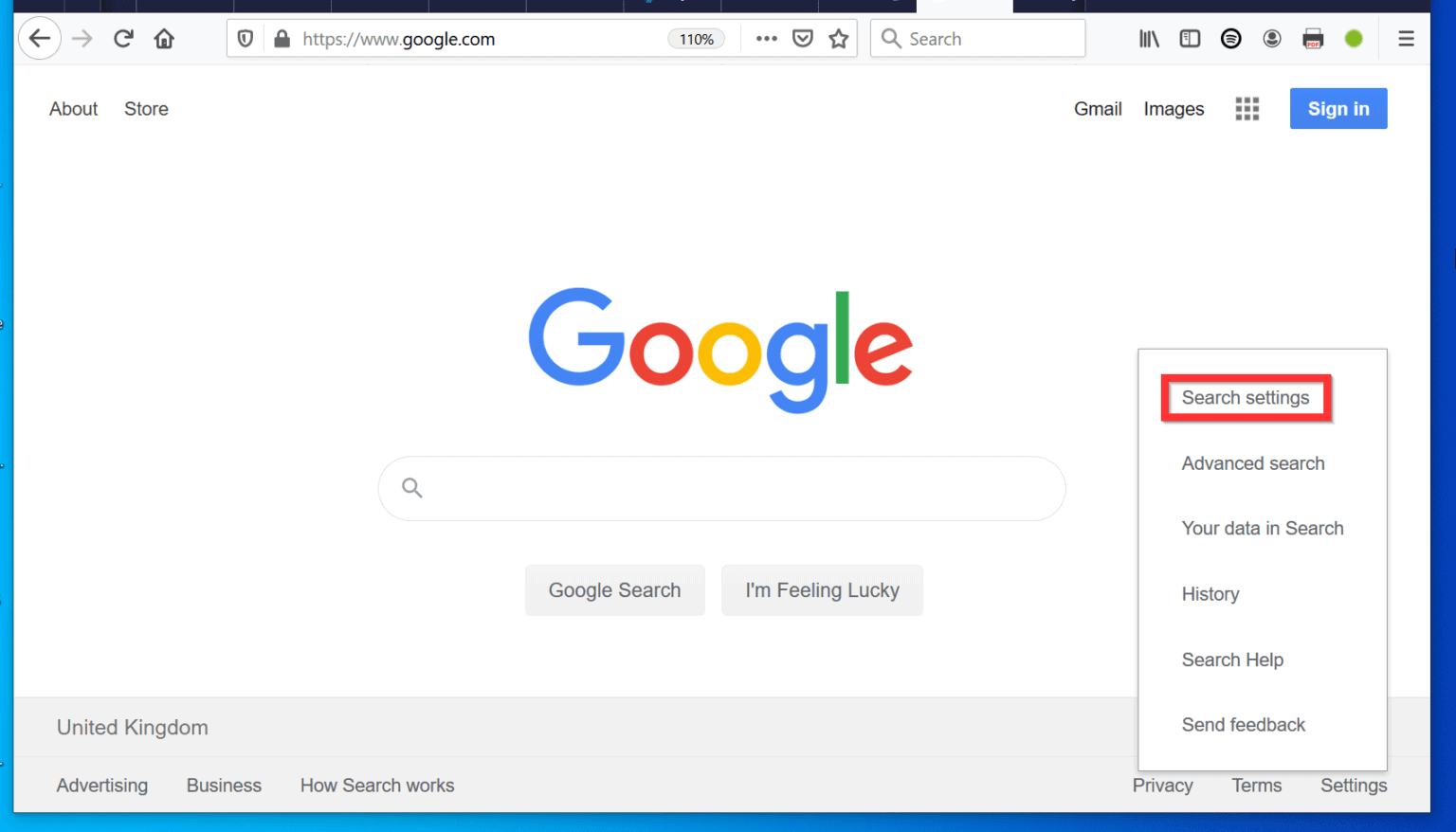The screenshot displays a web browser interface against a white background. The right edge features a dark blue vertical line that transitions to a sky blue color toward the bottom. Similarly, the left edge and top border showcase a sky blue hue and a thick black line, respectively.

In the upper left corner, there is a left arrow icon button, followed by a right arrow button, and then a reload button labeled 'Home.' Next to these buttons is a search bar adorned with a shield icon and a lock icon. Within the search bar, the URL "https://www.google.com" is displayed in gray text, except "google.com," which appears in black text. To the right of the URL, a small gray oval contains the text "110%" in black.

Further to the right are three dots arranged vertically, signifying an ellipsis, and a shield icon followed by a star icon. Adjacent to these icons is another search bar featuring a magnifying glass icon and the word "Search" on the left side. The right side of this search bar includes icons for a printer and a green circle. Additionally, three horizontal lines indicating a menu are located on the far right.

Below these elements, there are three lines of black text on the left side: "About" and "Store." On the right side, bolded text reads "Gmail" and "Images," followed by a grid of squares icon and a blue "Sign In" button with white text.

Centered beneath these features, the Google logo is prominently displayed, accompanied by a Google search bar. Below the search bar are two gray buttons: "Google Search" on the left and "I'm Feeling Lucky" on the right.

Near the bottom right corner of the screen, a gray-outlined rectangle encloses a list of options: "Search settings," "Advanced search," "Your data in Search," "Search history," "Search help," and "Send feedback." Notably, "Search settings" is highlighted with a thick red outline.